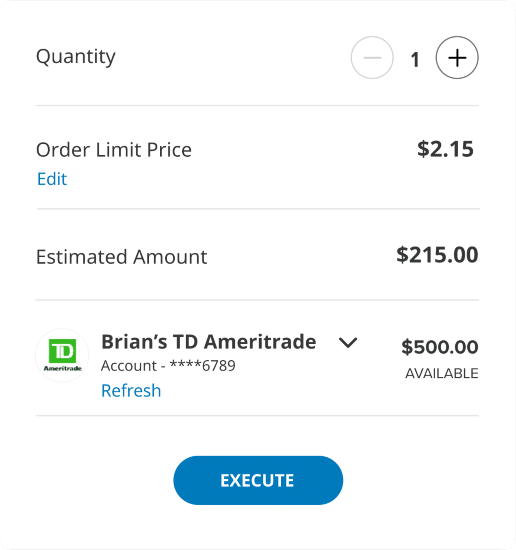The image appears to be a screenshot taken from either a phone or a computer, displaying an order form interface. At the top of the screen, there's a section labeled "Quantity" with a minus and plus button on the right side, and the current quantity set to 1. Below that, there's an "Order Limit Price" section, with the word "Edit" in blue on the left and a price of $2.15 on the right.

Further down, the "Estimated Amount" section shows a total of $215 to the right. At the bottom, there is a green square labeled "TD," next to text that reads "Brian's TD, American Trade Account," followed by an account number partially obscured with asterisks: ****6789. A drop-down option is available for selecting a different account, with a "Refresh" button in blue underneath. To the right of the available balance, it indicates $500. At the very bottom of the screen, a blue oval-shaped button labeled "Execute" completes the interface.